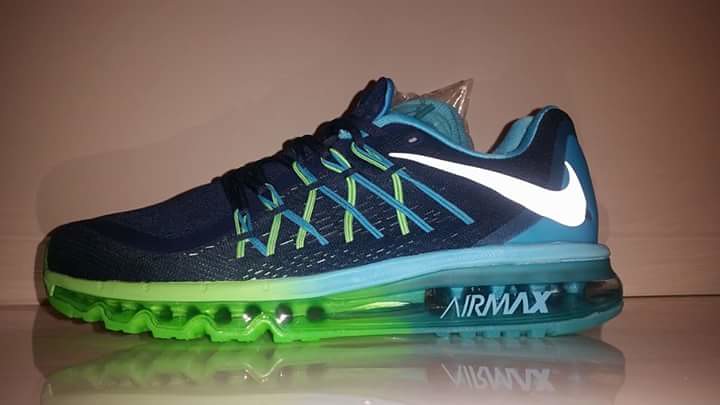This up-close photograph features a detailed view of a Nike Air Max tennis shoe. The shoe is oriented left, showcasing its side profile against a white, slightly grayish wall with a gray trim at the bottom, likely taken indoors. The shoe sits on a reflective surface, capturing a clear reflection beneath it.

The Nike Air Max boasts an intricate color gradient. Starting at the front, the sole is green, transitioning to turquoise, then bright blue, before softly fading into teal at the midsection, where it reads "Air Max" in white lettering. The jagged and bumpy rubber sole features spaced-apart columns, matching the gradient of the sole.

The shoe is predominantly blue, with variations from dark blue at the back to a lighter blue towards the front. The fabric comprises a blue mesh netting, transitioning to a lighter blue around the rear. White accents include the iconic, reversed Nike swoosh towards the heel and a strip on the sole. The laces are a mix of green and blue, adding to the vibrant palette. Notably, extra laces are tucked inside the shoe, which is padded for display purposes.

The overall sharpness and clarity of the photograph highlight the contemporary design and fresh look of the Nike Air Max, with no signs of wear, emphasizing its modernity and style.